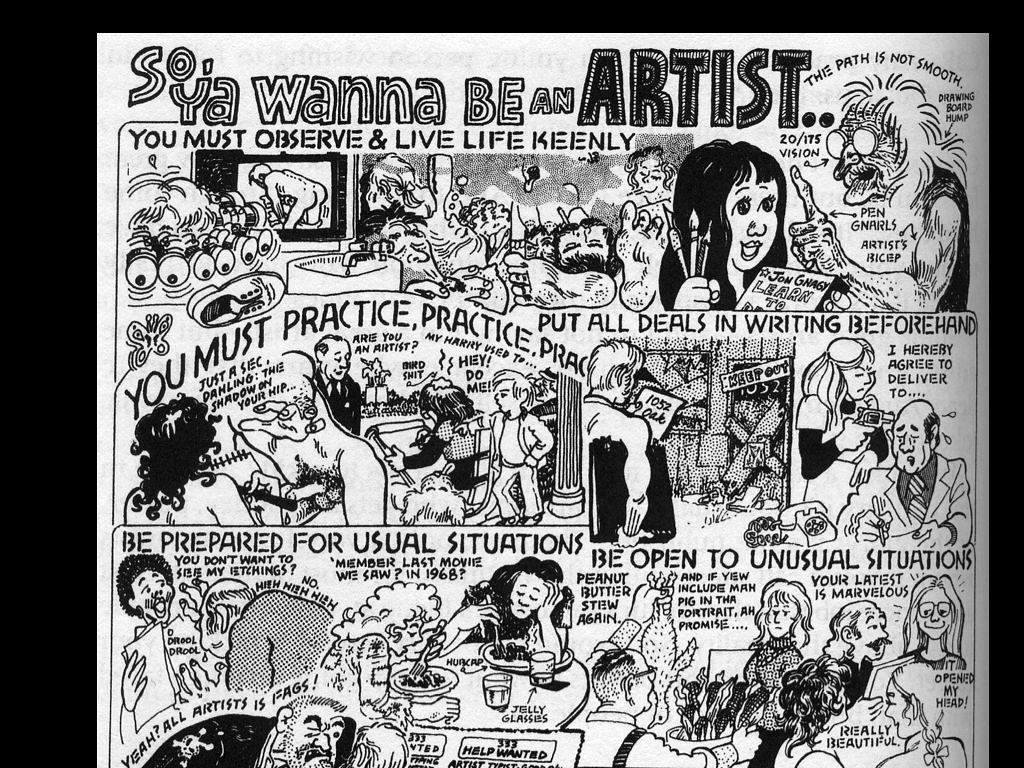The image is a hand-drawn, black-and-white comic strip titled "So You Want to Be an Artist?" It consists of multiple panels, each exploring the challenges and insights of an artist's journey. The comic emphasizes several key messages: 

- **Observing and Living Keenly:** The top of the image declares, "You must observe and live life keenly," accompanied by a bizarre creature with multiple eyes and a naked man bent over in water.
- **Practice Diligently:** Another panel insists, "You must practice, practice, practice," showing a naked man and woman, with the man commenting on the shading technique, "Just a sec, darling, the shadow on your hip."
- **Be Prepared and Open:** Further panels advise, "Be prepared for usual situations. Be open to unusual situations," illustrating the unpredictable and varied experiences one might encounter. There are scenes of people in everyday activities: a lady eating breakfast with her hand on her head, a girl drawing in a park with a young boy observing her, and random characters engaged in conversations and arguments.

Scattered amidst these illustrations are snippets of advice on practical preparation, such as, "Put all deals in writing beforehand," with a cartoon showing a woman next to a man with a telephone saying, "I hereby agree to deliver."

The comic's artwork is intricate and detailed, filled with strange and diverse drawings that together depict the multifaceted and often challenging life of an artist. The writing overlays the images, at times becoming small and less readable, reinforcing the notion that an artist's path is not straightforward or easy.